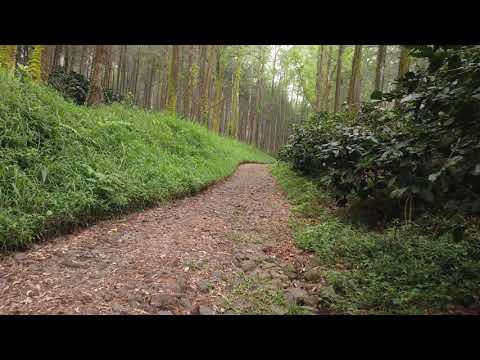This daytime image captures a serene forest scene with a centered walking path made of gray rocks, brown dirt, wood chips, and occasional leaves, extending vertically through the middle of the frame. The path is surrounded by natural elements: to the left, a gentle incline covered in thick green grass leads up to several tall trees with visible trunks adorned with patches of moss; to the right, there's dense brush and darker green bushes. The top of the image is dominated by the upper portions of these trees, though a few visible leaves hint at their height. It's a clear point-of-view shot, possibly taken by someone enjoying a walk through this tranquil natural setting. The overall color palette includes varying shades of green from the grass and bushes, browns from the pathway and tree trunks, and tans and white specks adding texture to the dirt pathway. The scene is text-free and person-free, emphasizing the peaceful, untouched environment.